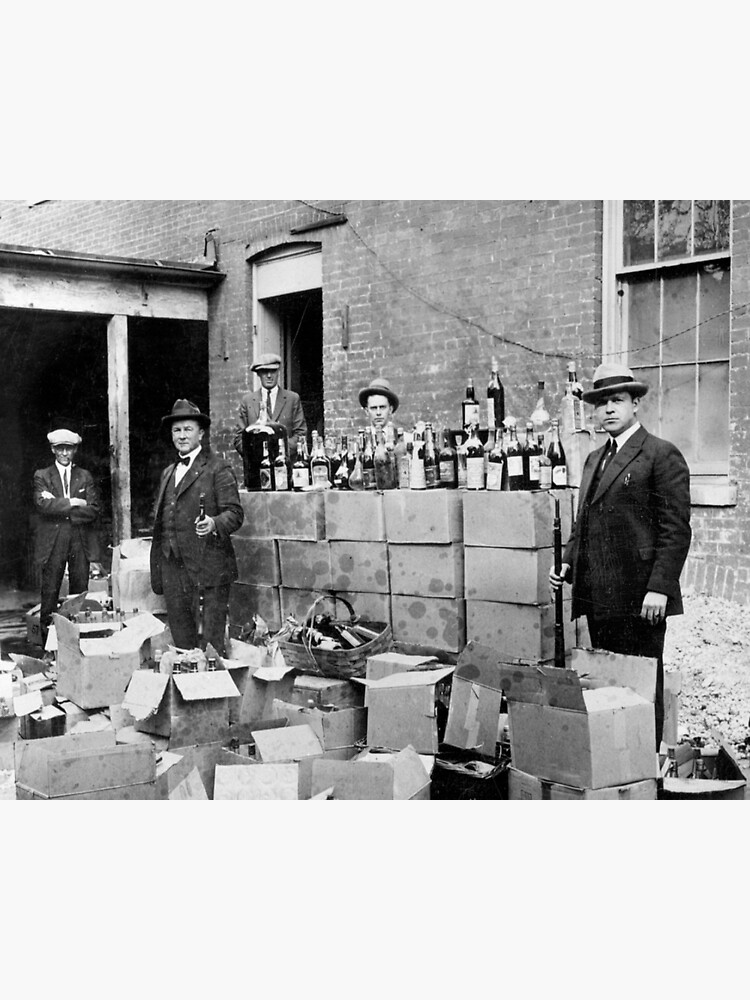In this black and white photograph, we find a group of men from what appears to be the 1930s or 40s, likely involved in a bootlegging operation. The image, though slightly grainy, is detailed enough to show that they are standing in front of a dilapidated brick building, which resembles a warehouse with obscured windows. The men, dressed in suits, ties, and various styles of hats (including brims and caps), are positioned around stacks of cardboard boxes filled with liquor bottles. Some of these boxes are open, prominently displaying brown and clear bottles of what seems to be moonshine. In the foreground, a basket also filled with liquor bottles adds to the display. One man wields a rifle, another holds a pistol, and yet another appears to hold a club. The scene, reminiscent of an illegal alcohol operation, captures a gritty slice of history marked by prohibition and the underground liquor trade.